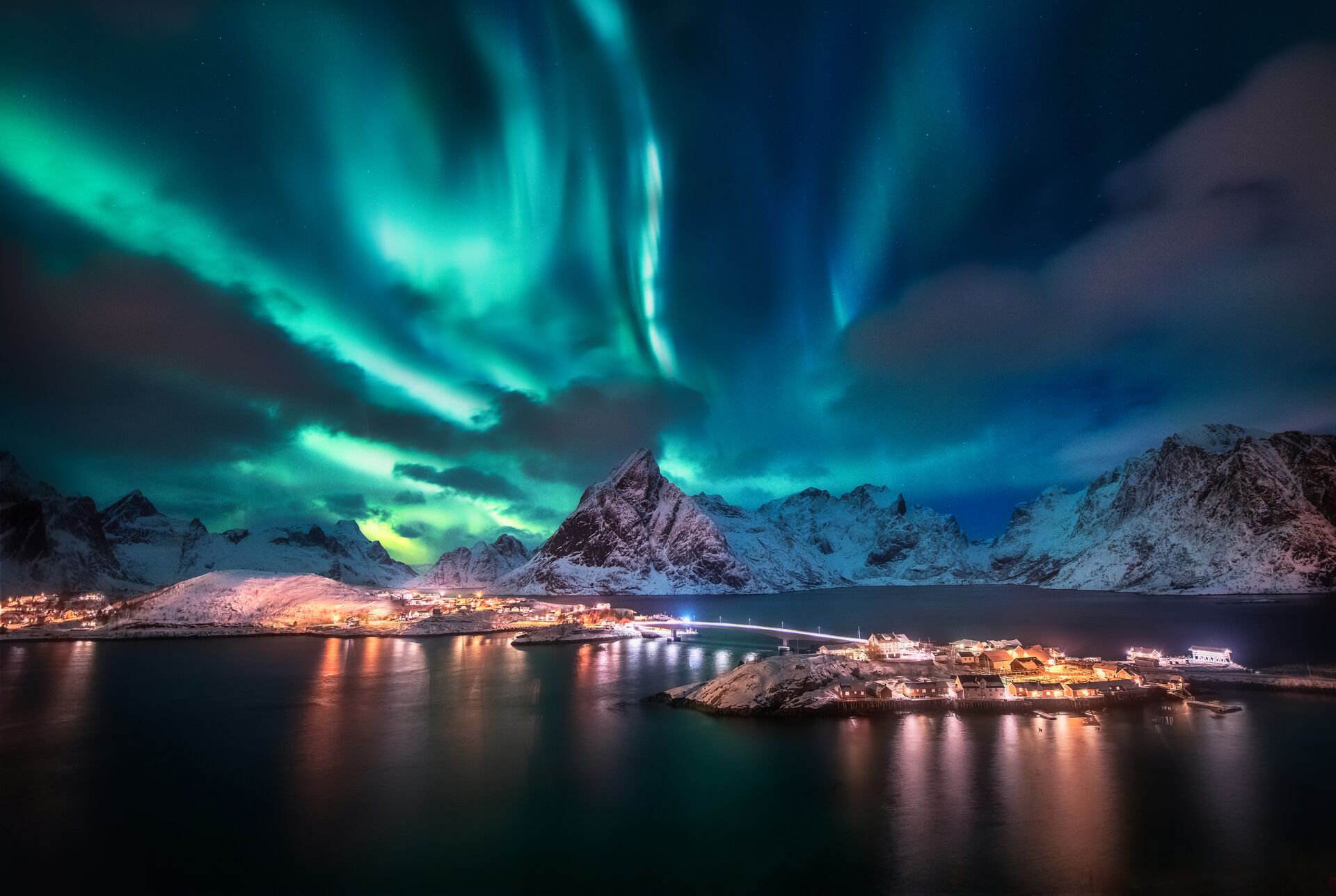In this visually striking image, the dark night sky is illuminated by the mesmerizing waves of the Aurora Borealis, also known as the Northern Lights, which stretch from the middle to the upper portion of the scene. The sky's deep blue hue is accentuated by sharp, luminous streaks of light and is interspersed with numerous clouds, creating a dynamic and captivating atmosphere. The landscape below features towering, snow-capped mountains that span from left to right, separating the celestial display above from the human elements below.

Nestled in the foreground, a small island-like area is visible, surrounded by still water. This island area hosts a collection of dwellings and buildings, each emitting warm, inviting lights that suggest occupancy and activity. A bridge connects this island to the mainland, adding an architectural element that bridges nature and civilization. To the left of this settlement is a larger city area, which also has buildings illuminated against the darkened sky. The entire scene combines natural and man-made beauty, portraying a serene yet vibrant nocturnal landscape.